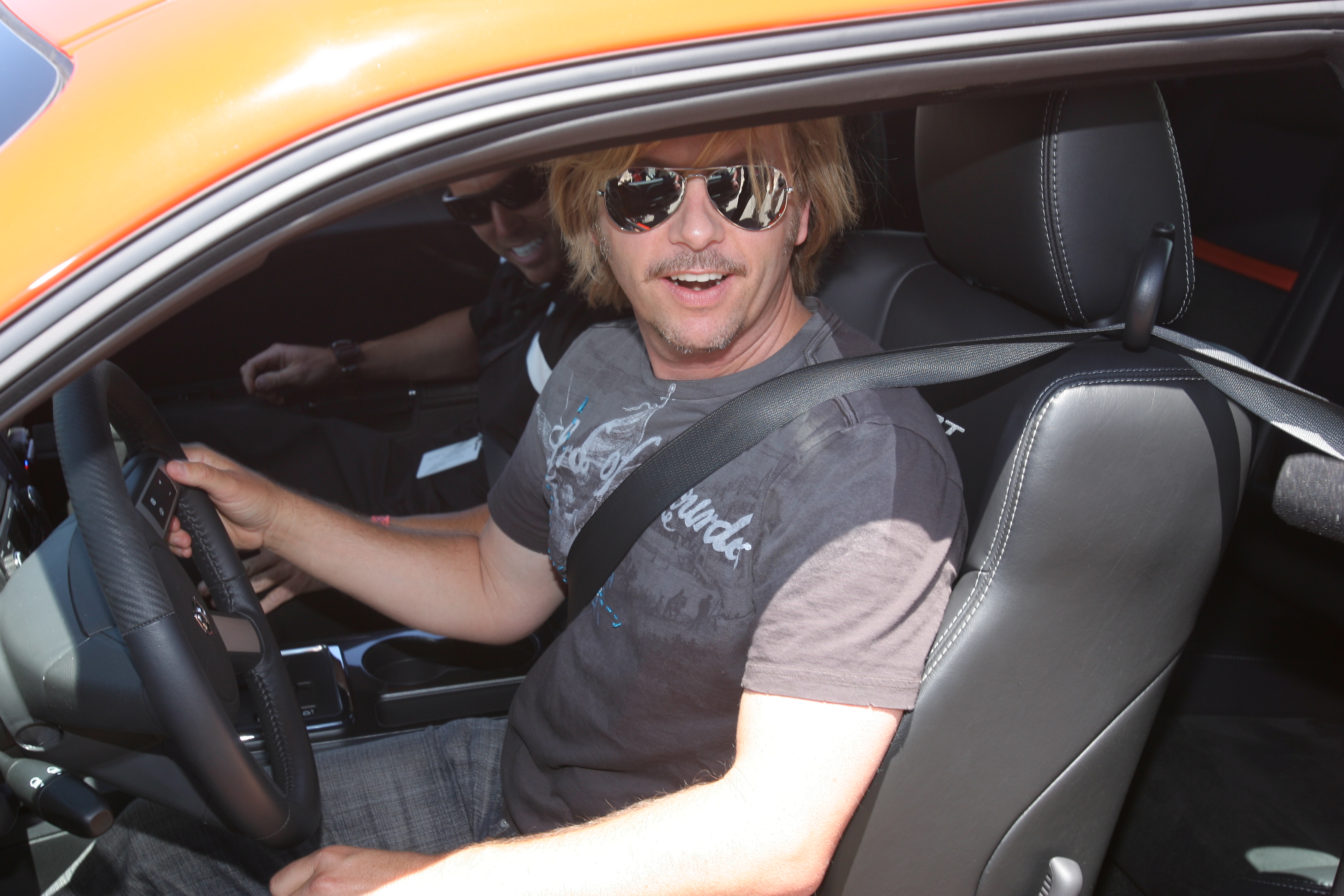In this vibrant photograph, comedian and actor David Spade is captured in an orange muscle car, exuding a relaxed yet cool demeanor. Spade, donning a black t-shirt, gray pants, and sunglasses, is seated in the black driver's seat, secured by his seatbelt. His signature short, flyaway blonde hair frames his face as he appears to be in mid-conversation, his mouth open in a casual smile. Beside him in the passenger seat is another man, also sporting sunglasses and dressed in black, who closely resembles Ryan Reynolds. This individual is slightly faded in the background but adds a recognizable presence to the scene. The car's gray interior complements its striking exterior, visible through the angle capturing mostly the driver's side and hinting at the back seat. The photograph offers a dynamic snapshot of the two men enjoying a moment in the stylish, presumably beloved, muscle car.